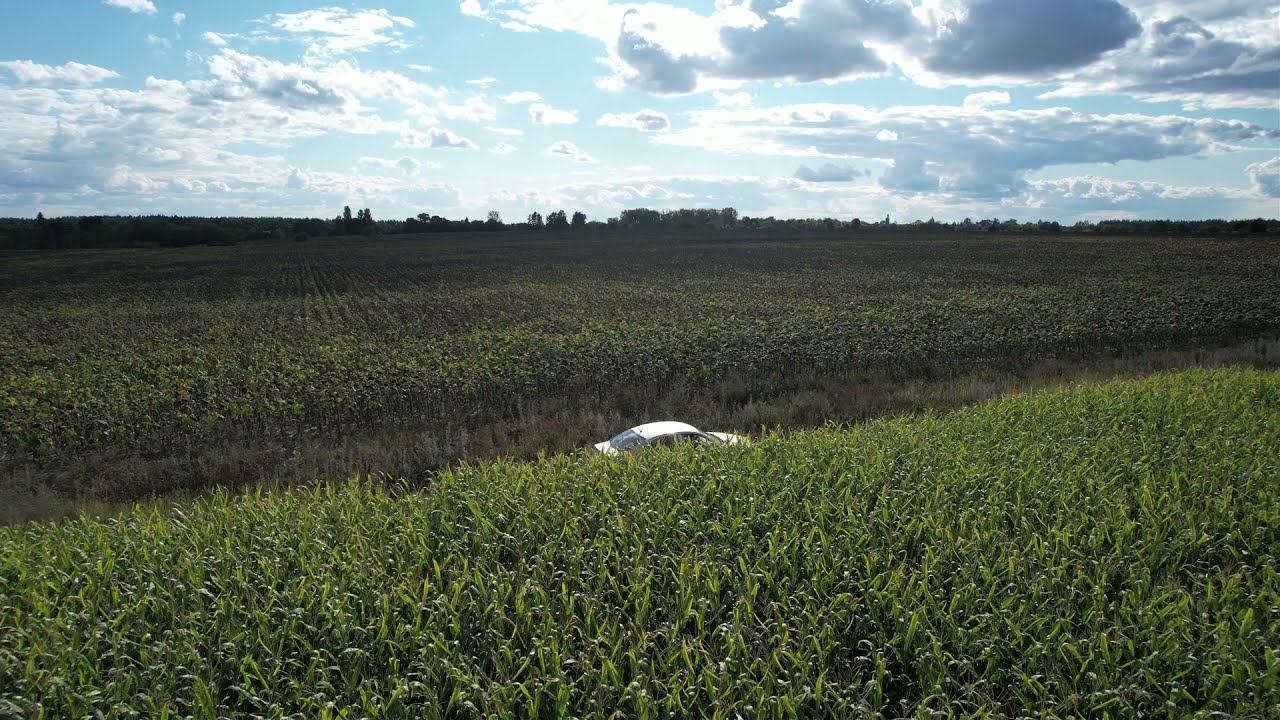The image captures a drone's-eye view of a lone white sedan driving through a path that cuts through expansive farmland, possibly a cornfield with tall, green crops that have not yet begun to bud. Although the road itself is not visible, the gap in the crops clearly indicates its presence, with lush greenery on either side of the vehicle. Occupying the bottom two-thirds of the image, these undulating fields lead the eye toward a distant tree line silhouetted against the sky. The top third of the photograph reveals a pale blue sky, with heavier, more clustered clouds on the right side and sparser clouds on the left, casting soft shadows over the landscape. The scene is a blend of realism and photographic representationalism, accentuated by the natural light and shadow interplay, characteristic of landscape photography.